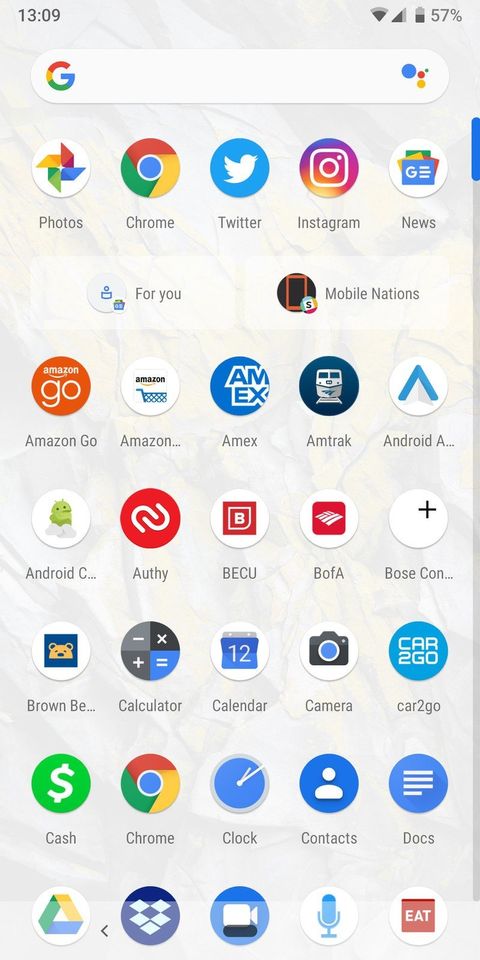The image showcases the app drawer of an Android phone, set against a background that appears either light silver or semi-transparent, revealing a rocky, ancient terrain-like wallpaper beneath. At the top of the screen, a selection of frequently used apps is separated from the rest, suggesting these may be favorite or docked icons. These include Photos, Chrome, Twitter, Instagram, News, and two unique buttons labeled "For You" and "Mobile Nations." Below, the main app drawer unfolds in alphabetical order, starting with apps like Amazon, Amex, Amtrak, Android Auto, Authy, B of A, Calculator, Calendar, and Camera. The multitude of apps extends well beyond the initial screen, reaching up to the beginning of the 'E' section, indicative of a vast collection. A search bar sits at the top for easy navigation, while the status bar reveals the phone is at 57% battery and set to 24-hour time, displaying 13:09.